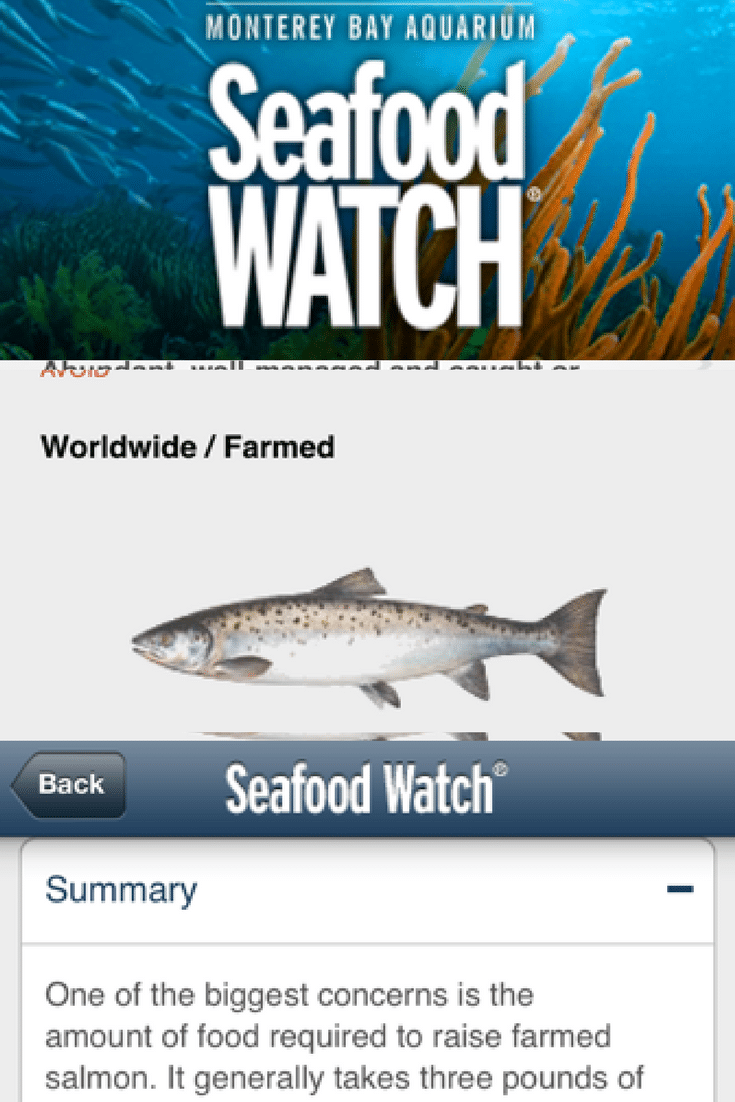This image is a promotional display from the Monterey Bay Aquarium, advertising their Seafood Watch program. The poster showcases the initiative's focus on globally sourced farmed seafood. At the center of the image is a life-like fish set against a vivid underwater backdrop. To the left, there's a dynamic school of fish, and a vibrant coral reef stretches across the background, with splashes of orange contrasting against the deep blue waters on the right. Unfortunately, the very top of the advertisement is partially cut off. Below the central fish image, there is a black "back" button with "BACK" written in white. The text under this button reads "Seafood Watch," followed by a brief summary highlighting sustainability concerns: "One of the biggest concerns is the amount of food required to raise farmed salmon. It generally takes three pounds of," which is unfortunately cut off, leaving the rest of the sentence unreadable.